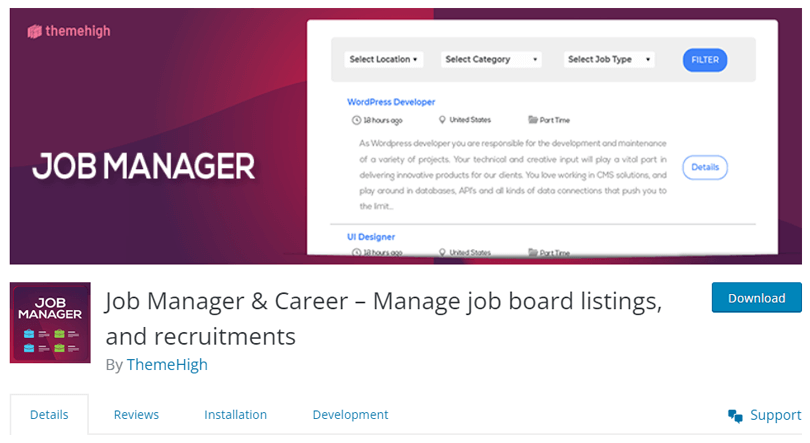The image features a rectangular purple box that transitions to a lighter purple shade towards its center. In the top left corner, the text "Theme High" is displayed in pink. Below that, the words "Job Manager" are prominently written in large white capital letters. Positioned within the purple box is a white rectangle containing three drop-down menus labeled "Select Location," "Select Category," and "Select Job Type." Next to these menus is a blue button labeled "Filter."

Beneath the filter options, the text "WordPress Developer, 12 hours ago, United States, Part-Time" appears. Further below, there is a job description for a WordPress Developer, stating that the role involves the development and maintenance of various projects. The description emphasizes the importance of the candidate's technical and creative input in delivering innovative products for the company's clients. Additionally, the job involves working with OHS Solutions, database management, and handling diverse data connections.